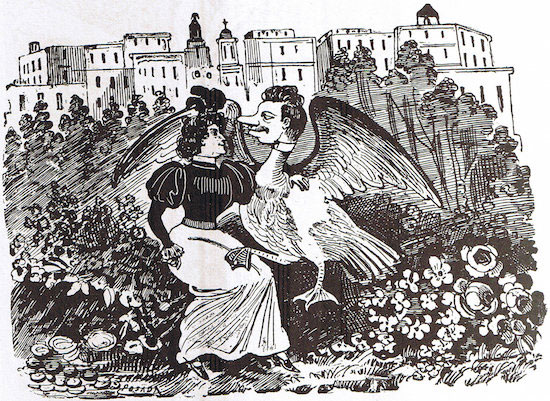This wide, rectangular artwork, created in black and white on light gray to white paper, appears to be rendered with bold black ink or pen lines. The composition includes a simplistic cityscape in the background, featuring tall rectangular buildings with thin, vertically-oriented windows. Some structures are adorned with bells and crosses, suggesting churches, evoking a late 1800s or early 1900s European setting. In the foreground, there are clumps of green trees, bushes, and scattered white flowers, adding to the scene's lushness.

Prominently seated in the center foreground is a woman dressed in period attire, wearing a thick black top with poofy sleeves and a long white skirt that reaches her ankles. She has curly black hair and is engaged in an intriguing interaction with a fantastical bird-like creature with the head of a man. This creature, featuring a large nose, a mustache, and short curly black hair, sports a collar around its neck. Its body, resembling that of a duck with widespread wings and webbed feet, adds an element of surrealism to the scene. The man-bird's right foot rests delicately on the woman's lap as they share a moment, looking at each other amidst the detailed foliage and historical backdrop.